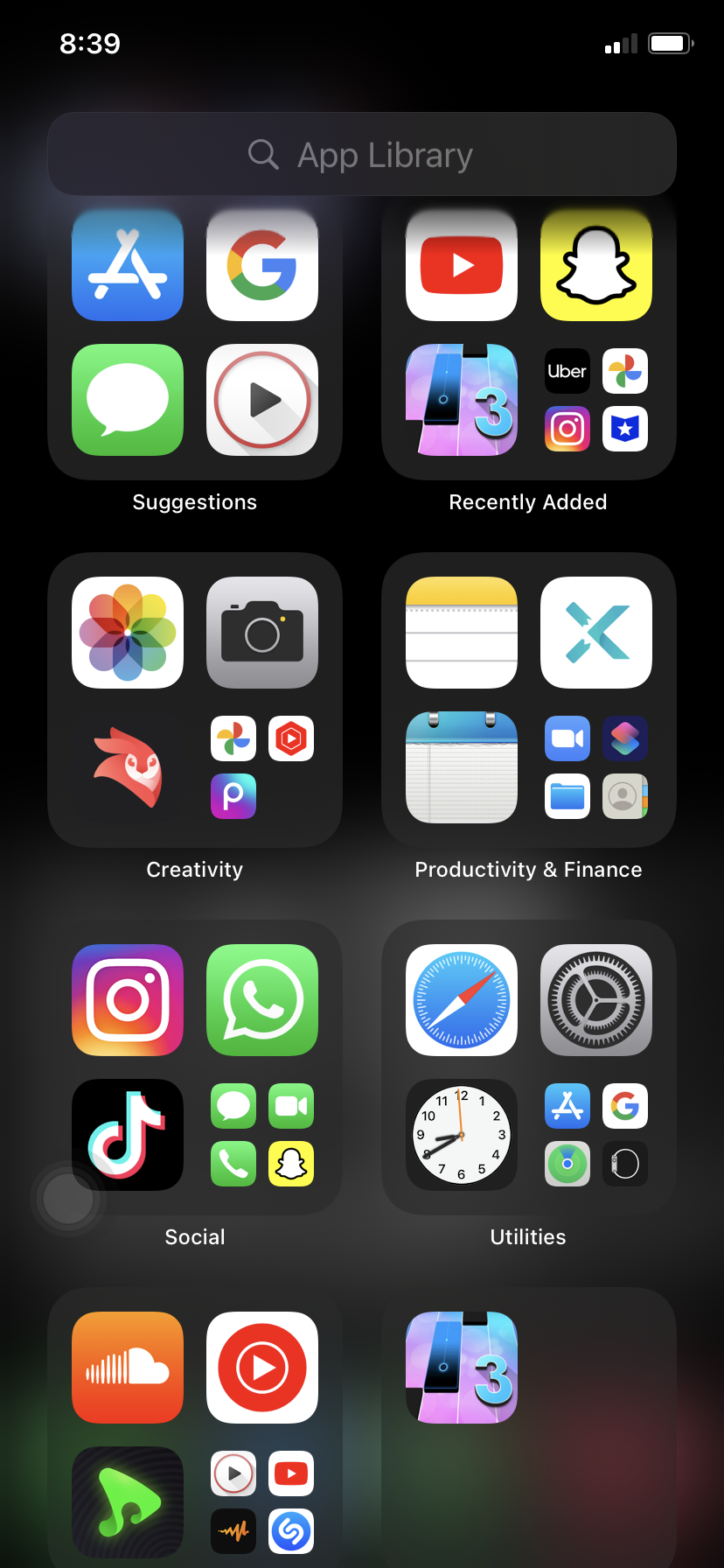The image is a screenshot of a smartphone displaying various apps organized in a folder-style layout against a background that transitions from black to gray, with hints of green and red near the bottom. The top left corner shows the time as 8:39, and the top right corner indicates two out of four bars of signal strength and a nearly full battery. At the top, a grayed, oval-shaped search bar with a magnifying glass icon reads "App Library."

The first section is labeled "Suggestions" and features the icons for Google, a messaging app, a red circle with a play button (likely YouTube), and an "A" on a blue background. Below, the "Recently Added" section includes YouTube, Snapchat, Uber, and Instagram icons.

The "Creativity" section displays icons for camera and Photoshop apps, while the "Productivity and Finance" section includes various spreadsheet programs. The "Social" section features icons for Instagram, TikTok, and WhatsApp. The "Utilities" section shows icons for Compass, Clock, and a gear symbol for settings.

In the bottom left corner, the "Music" section includes icons for Shazam, SoundCloud, and another app with a red bullseye and play button, possibly indicating another music-related application.